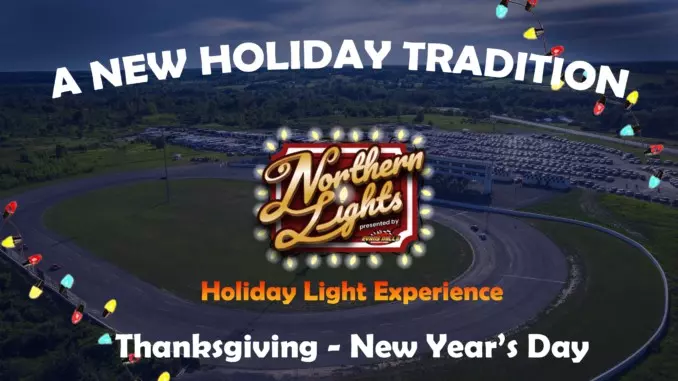This advertising poster, predominantly in dark blue, features a compelling aerial view of an oval racetrack with a vast green lawn at its center. The poster accentuates the holiday spirit with festive Christmas lights strung across the lower left and upper right corners. At the top, in white lettering, the text reads "A New Holiday Tradition." Central to the design, a marquee-style lighted perimeter frames key event details: "Northern Lights, Holiday Light Experience." The Northern Lights logo boasts a vibrant red background with yellow lettering, while "Holiday Light Experience" shines in an amber or orange gradient. Below, the timeframe "Thanksgiving through New Year's Day" is clearly noted. The racetrack itself is subtly lit with colorful lights—blue, yellow, and red—peppering the lower left section. Additionally, a small, indiscernible logo is mentioned as the presenter. In the backdrop, a parking lot filled with cars adds a layer of realism, underscoring the event's anticipated popularity.